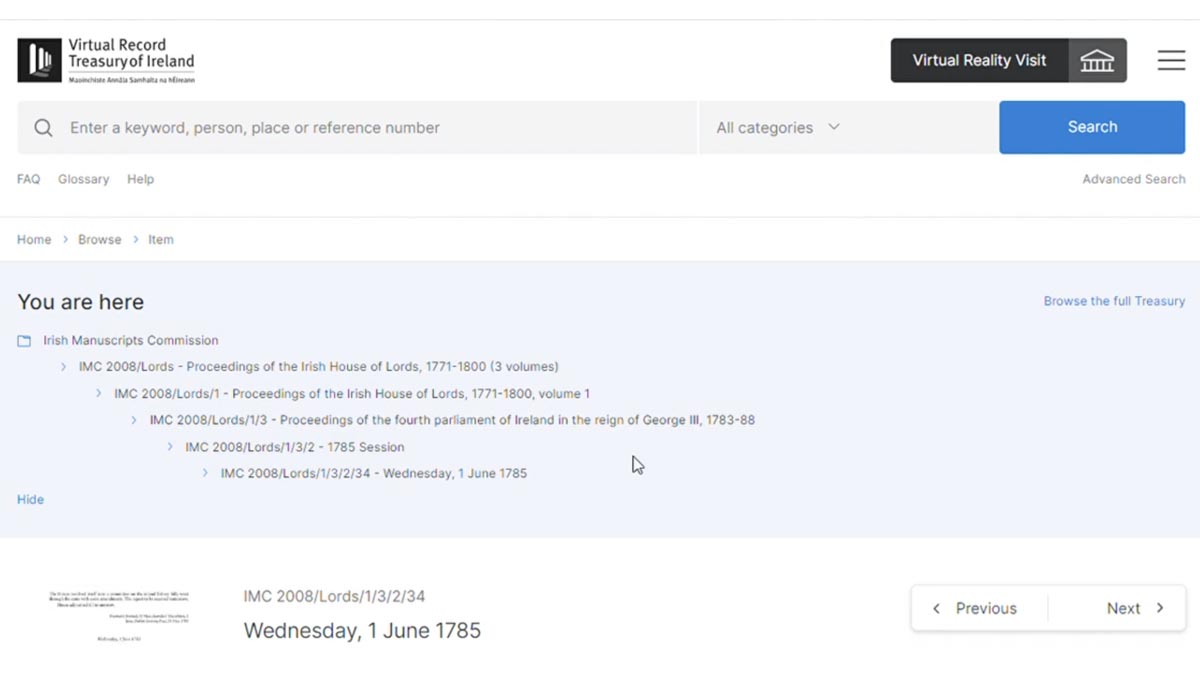The image showcases a detailed interface with multiple sections. 

**Top Section:**
- A thin gray line spans the width of the image against a white background.

**Center Section (Left to Right):**
- A square with a black background features white vertical bars. Adjacent to this, the text "Red Roof Record" is written in black. Below this, the phrase "Treasury of Ireland" also appears in black.
- Another thin gray line separates this content from the next section.

**Lower Center Section:**
- Five small, indiscernible words appear, their details blurred when zoomed in.
- To the right, a rectangular, black background features the white text "Virtual Reality Visit." Accompanying this is a white building column icon and three gray lines beside it.
- Below this is a gray rectangular search box with a magnifying glass icon inside. The placeholder text in gray reads, "keyword, person, place, or reference number." Adjacent is a blue box with white text stating "Search."
- Following this, blue text reads "FAQ," while gray text indicates "Glossary Help.” Further right, "Advanced Search" is written.

**Bottom Section:**
- A thin gray line stretches horizontally.
- Beneath it, "Home" appears, followed by a blue arrow pointing to "Browse," with another blue arrow directing to "Item." 
- Alongside this is a light blue rectangular box with "Browse the Full Treasury" written in blue.
- Indicating the current location, text says "You Are Here," followed by "Ivory Manuscripts Commission" in black. 

**Footer:**
- Concluding the image, blue text reads "Hi," followed by "Wednesday, 1 June 1785" in black.

This meticulously layered interface likely pertains to an archival or historical database, complete with search functionalities, navigational aids, and indicators of current location within a repository.